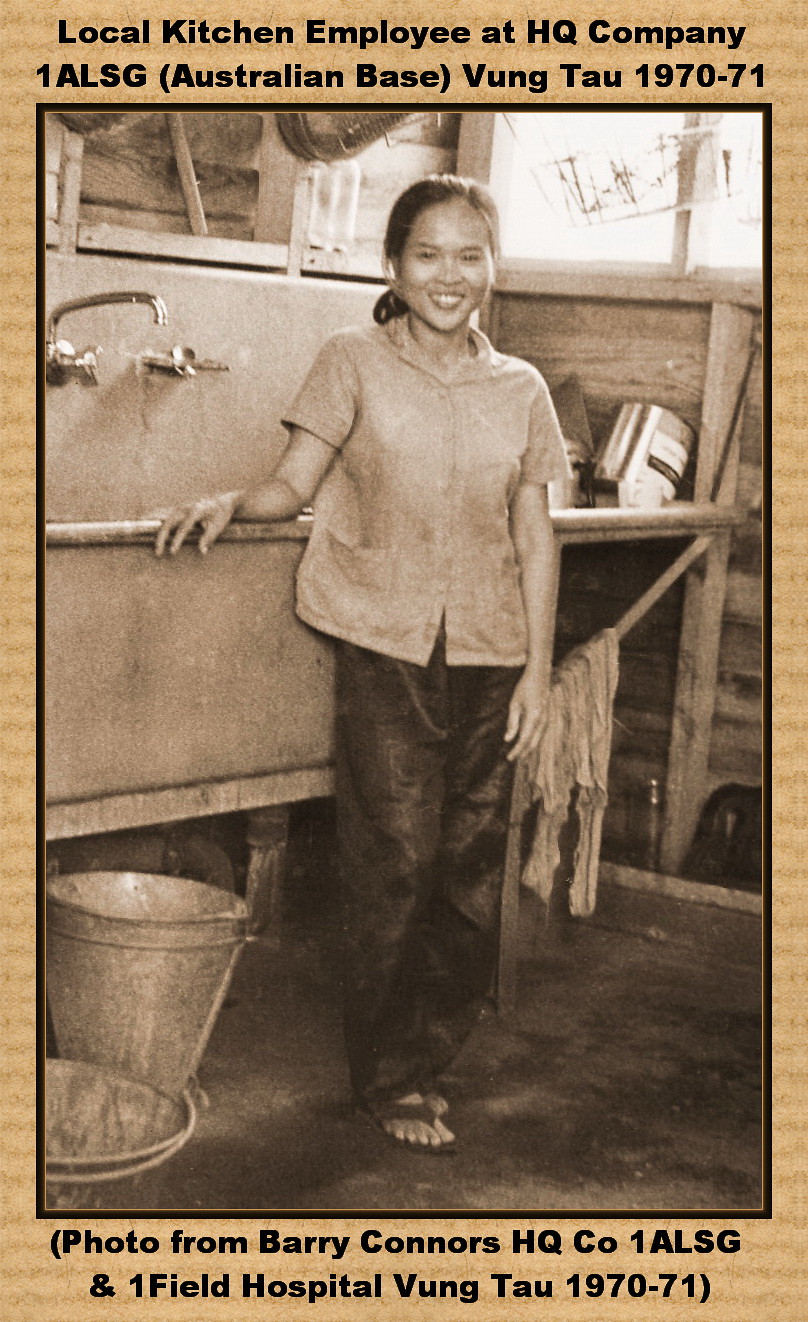The image features a vertically oriented black-and-white photograph framed by a tan corrugated cardboard border. At the top of the border, text reads, "Local Kitchen Employee at HQ Company, 1 ALSG, Australian Base, Vung Tau, 1970-71," and at the bottom, "Photo from Barry Connors HQ Company, 1 ALSG and 1 Field Hospital, Vung Tau, 1970-71." 

Centrally positioned is a short Vietnamese woman, possibly a girl, wearing a button-down short-sleeve blouse, black pants, and flip-flops. She is smiling directly at the camera, her hair neatly tied back in a ponytail. She stands in front of a large industrial-sized stainless steel sink, one typical of a mess hall or kitchen environment. Scattered around her are various objects, including a small metal bucket with its lid off, what appears to be paint cans inside the sink, and rags hanging on a nearby pole. The setting appears semi-outdoors, illuminated by daylight, suggesting it was taken during the day somewhere in Vietnam. The color palette includes shades of brown, black, tan, white, silver, and gray.